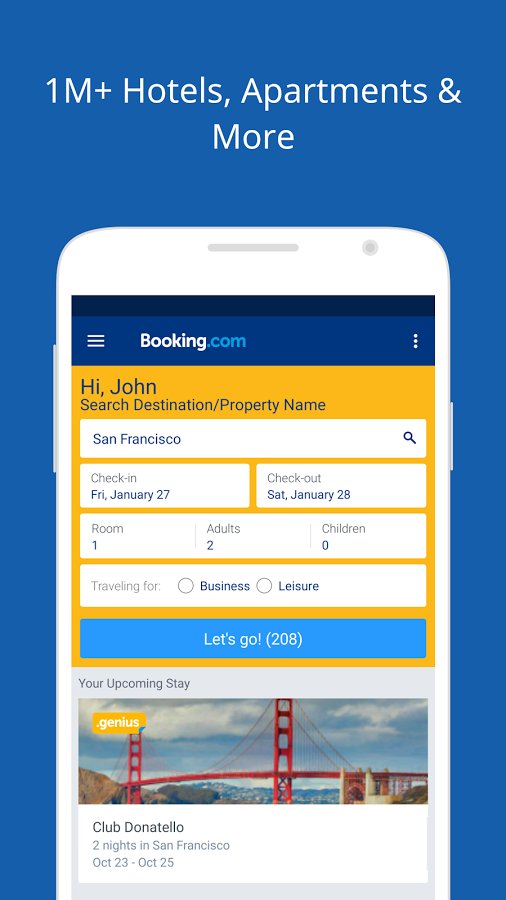In this detailed image, we see an advertisement for a mobile application, prominently featuring the Booking.com website displayed on a smartphone screen. The ad is primarily designed with a blue background and white text for high contrast and readability. At the top, the text announces "1 million plus hotels, apartments, and more," emphasizing the extensive offerings available through the app.

The smartphone display showcases the Booking.com interface, which greets the user with "Hi John" and includes a search bar for destination or property names. In this example, "San Francisco" has been entered as the destination. Below the search bar, several fields are visible: the check-in date is set for Friday, January 27th, and the checkout date for Saturday, January 28th. The reservation details further specify one room for two adults, with no children.

Additional options for selecting the purpose of the trip, either for business or leisure, are available. A prominent blue button labeled "Let's go" invites users to proceed with their search. The number 208, likely representing the count of available options, is also displayed.

Below these interactive elements, the ad includes information about an upcoming stay, featuring "Club Donatello," with a reservation for two nights in San Francisco from October 23rd to October 25th.

Overall, the ad effectively presents a clean, user-friendly preview of the Booking.com app, highlighting its functionality and ease of use for planning trips.